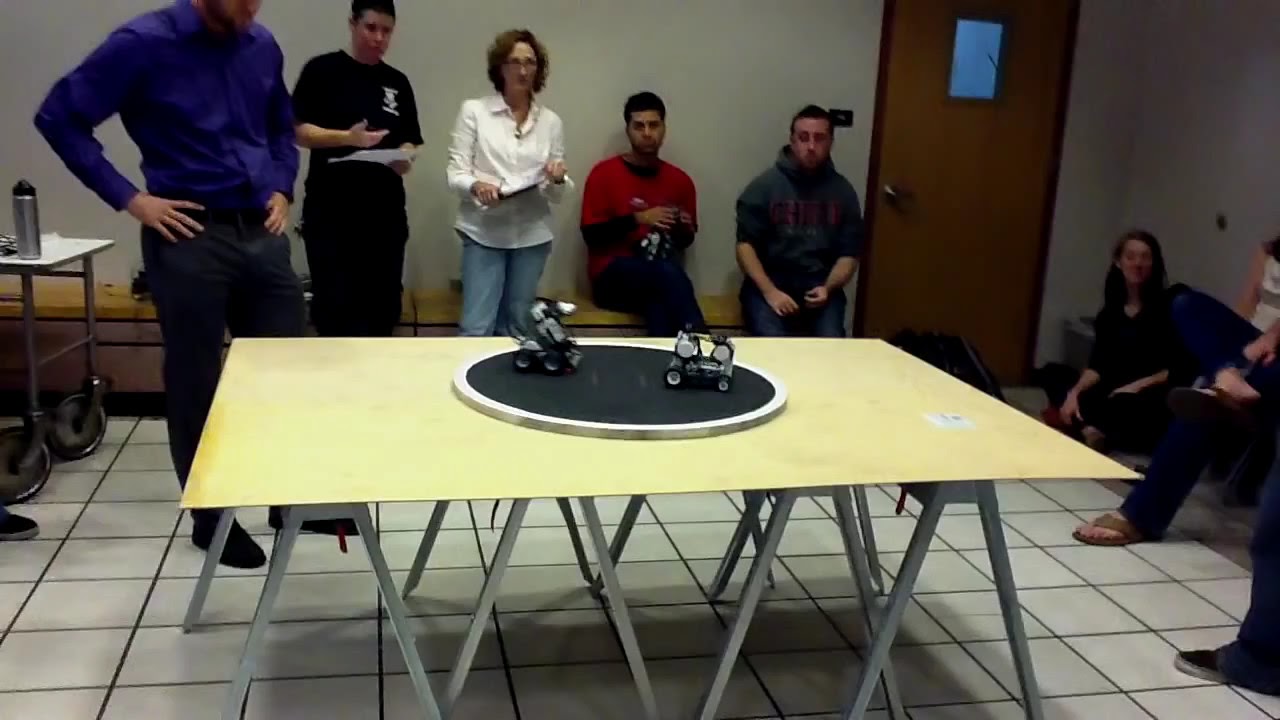This indoor, landscape-oriented color photograph captures a small group of people gathered around a makeshift table, set in a room with white walls and white square tile flooring with black grout. The light honey-colored plywood table is supported by four metal sawhorses and features a circular raised platform at its center, with a black center ring and an outer ring made of some silver metal. On the platform, there are two small, remote-controlled robotic vehicles, resembling Lego-like designs with wheels.

To the left of the table, a man wearing a blue jacket and black pants stands with his hand on his hips, though his face is slightly cut off at the top. Next to him is another man in a black t-shirt, holding a white paper and speaking. Toward the center stands a woman with glasses, medium-length brown hair, a white jacket, and blue jeans. To her left, two seated men watch the robots, with a door opening into the room beside them. On the right side, several people sit partially viewed, also observing the scene.

The room hints at a robotics convention or demonstration, engaging the attendees with the small robotic vehicles at the center of attention.